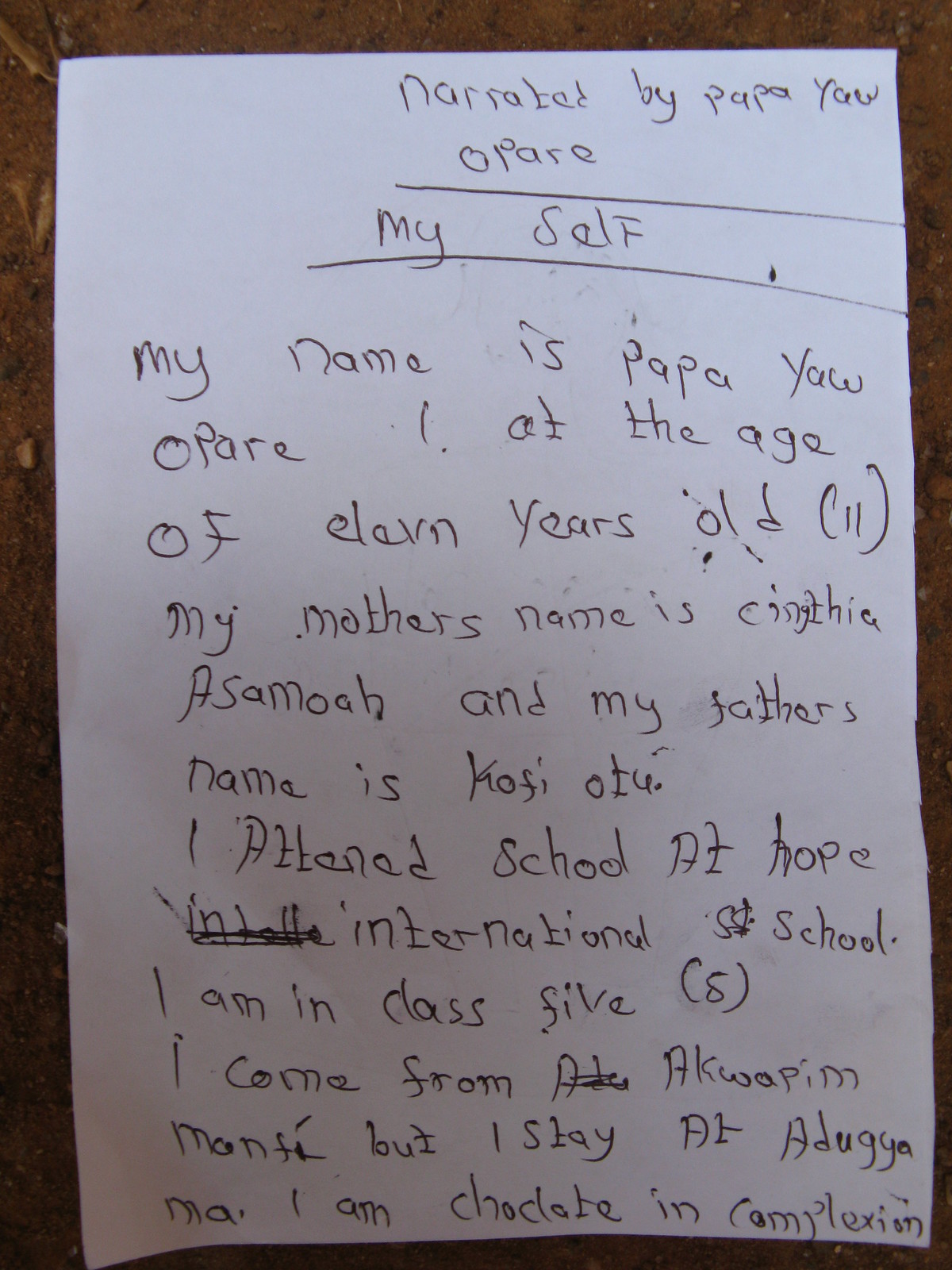The photo captures a handwritten note on a clean white sheet of paper placed on a brown surface. The note, titled "Myself," appears to be written by an 11-year-old named Papaya Opare. At the top of the note, it states "narrated by Papaya Opare." The note elaborates, "My name is Papaya Opare. I am 11 years old. My mother's name is Cynthia Asamoah, and my father's name is Kofi Otu. I attend Hope International School where I am in Class 5. I come from Akwapim, Monfi, but I stay at Adugwa Ma. I am chocolate in complexion." This depiction suggests that Papaya is likely a young African child.